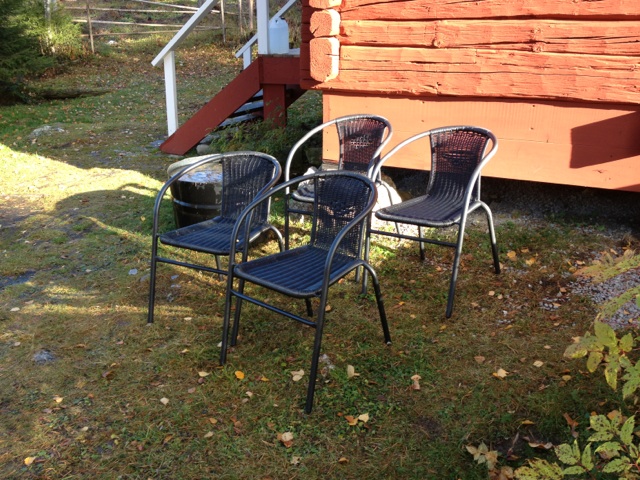The outdoor scene captures a quaint, rustic backyard dominated by a reddish log cabin or camp-style cottage. The house features a distinct red staircase with white railings leading up to it. The lush, light green grass is short and scattered with leaves, contributing to the serene, natural setting. In front of the house sit four chairs arranged in a row of two pairs, adding to the welcoming vibe. These chairs are predominantly black metal with woven material seats, likely rattan or black plastic, characterized by a unique looping design that forms both the armrests and the back legs. Adding to the cozy aesthetic is a large water basin, partially filled, positioned nearby. Visible in the lower right corner, a few leafy branches intrude, enhancing the sense of an inviting, verdant space.